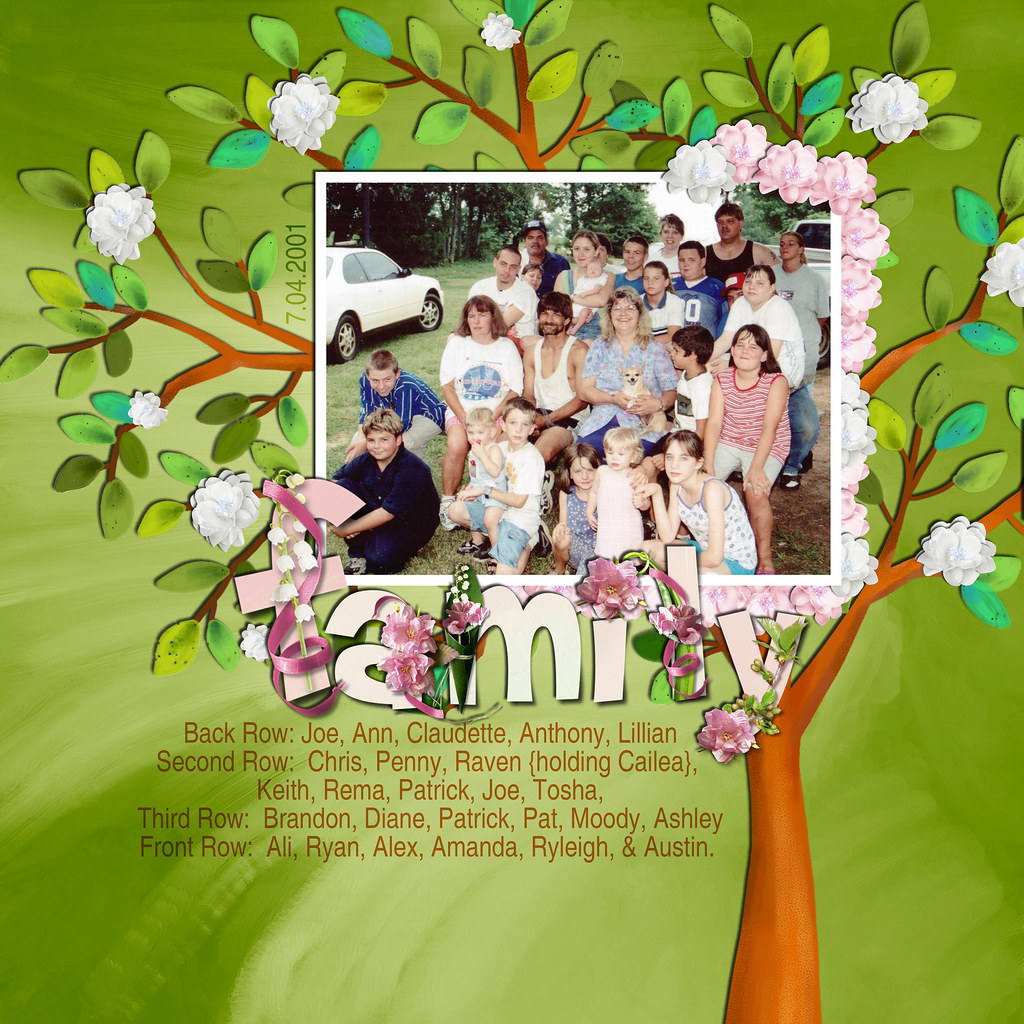The image showcases a meticulously crafted family poster featuring a large, multi-generational family photograph set outdoors. The central focus is on the family group, comprising approximately 30 members arranged in four rows according to height and age, with the youngest in the front and the tallest in the back. In the background, a beautifully illustrated tree with branches adorned with flowers extends across the composition, symbolizing the family tree. 

The photograph itself is framed with a white border embellished with flower petals on the right side and bottom. Below the image, the word "Family" is prominently displayed in large font, decorated with mixed media-style flowers and ribbons. The date "7.04.2001" is noted on the left-hand side, situating the moment in time. Underneath the decorative "Family" label, a detailed list of all family members' names is provided, organized by rows:

- Back row: Joe, Ann, Claudette, Anthony, Lillian
- Second row: Chris, Penny, Raven (holding Kalia), Keith, Rima, Patrick, Joe, Tasha
- Third row: Brandon, Diane, Patrick, Pat, Moody, Ashley
- Front row: Allie, Ryan, Alex, Amanda, Riley, Austin

This thoughtfully designed poster serves as a commemorative keepsake, capturing the essence and unity of the family.